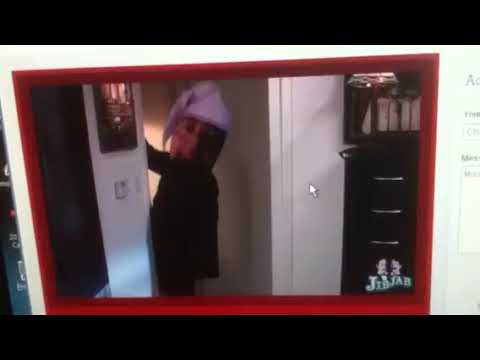The image is a rather unsettling screenshot from a JibJab video, displaying a figure with an oversized, blurry head superimposed onto a darkly dressed body. The head, which resembles a light brown mask or possibly a gingerbread man, looks disproportionately large and is adorned with a white, tassled cap akin to a Christmas or sleeping hat. The figure stands in a white doorway, partially entering a plain room with white walls and adjacent to black filing cabinets with visible handles. Behind the figure, you can see a dresser bathed in some light. The desktop of the computer screen is partially visible, along with a mouse cursor on the right and the cut-off interface of the JibJab video software, showing the logo and some text boxes. The image is framed distinctively in bright red, adding to its peculiar and eerie ambiance.